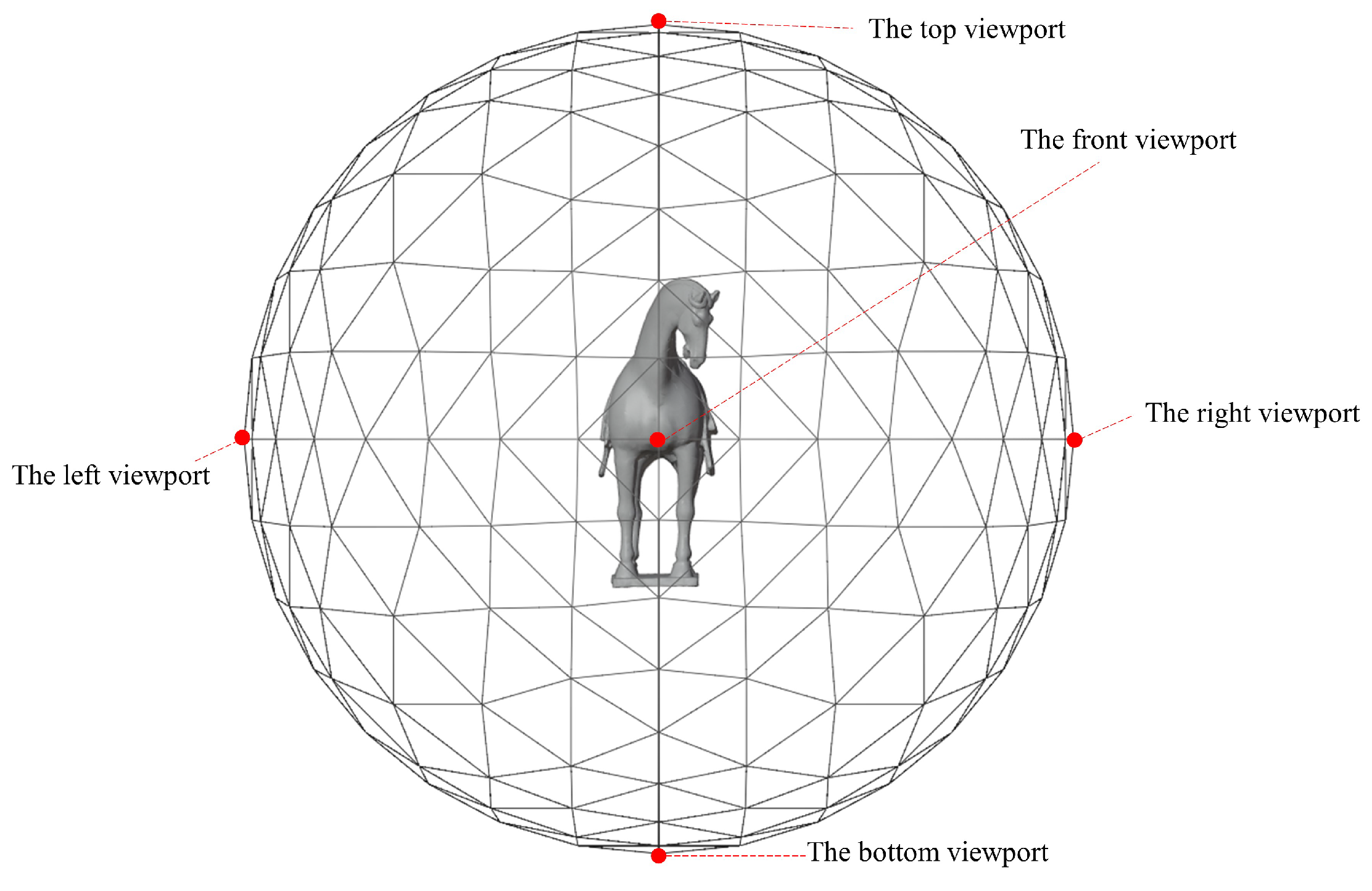The image is a detailed digital diagram featuring a transparent, highly faceted sphere composed of numerous intersecting triangles, creating a mesh-like structure. The sphere is set against an all-white background, allowing clear visibility of its contents. Inside this sphere, centrally located, is a grey, 3D-rendered horse viewed from the front. The horse appears to be made of plastic and strikes a pose with its head slightly tilted downwards to its right.

The diagram includes several labels connected by red lines that end in small red dots positioned at specific locations on the sphere. These labels identify different viewports: "Top Viewport" at the top, "Bottom Viewport" at the bottom, "Left Viewport" on the left, "Right Viewport" on the right, and "Front Viewport" in the center. The red lines and dots highlight the corresponding points on the sphere, enhancing the visual understanding of the various viewports within this intricate digital rendering.